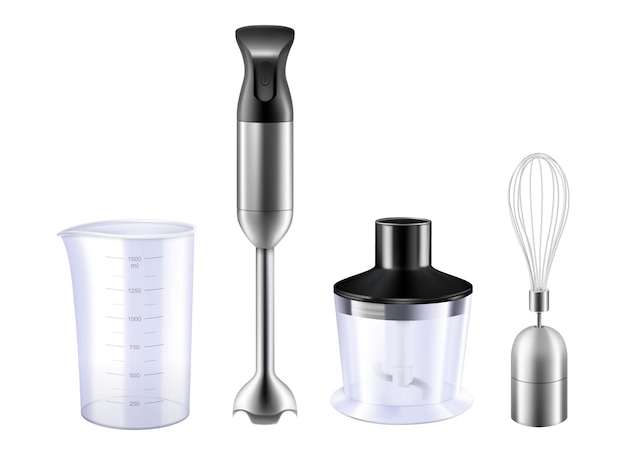This image showcases a set of sleek, contemporary kitchen gadgets against a pure white background. Starting from the left, there is a clear measuring cup with a spout and measurement lines ranging from 250 mL to 1,500 mL. Next is a stainless steel hand blender with a black handle and a silver base, featuring a smooth, bladeless design. To its right is an automatic food chopper with a clear plastic container and a black lid, suitable for small food items. Lastly, there is a silver whisk attachment with a metal half-bullet shaped connector, designed to be attached to the hand blender for whisking tasks. All items are pristine and presented in an orderly fashion, emphasizing their functional and aesthetic appeal.